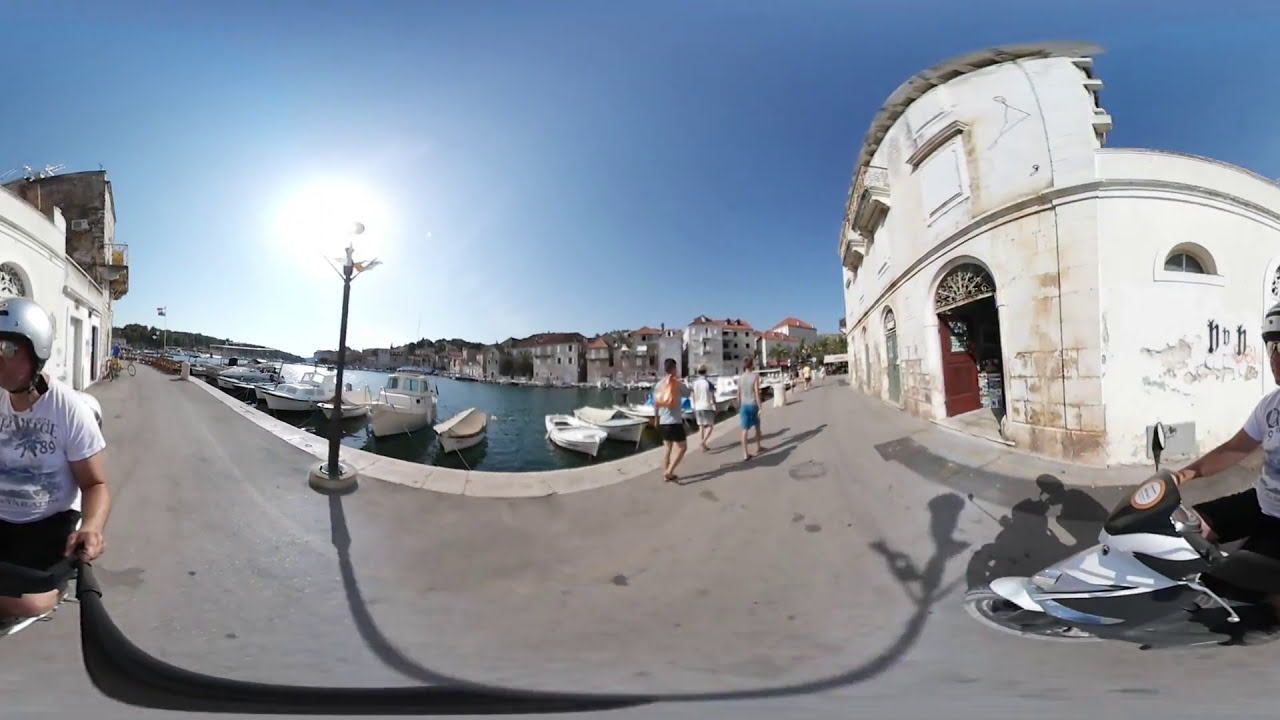In this vibrant and somewhat distorted outdoor photograph, you are gazing at a picturesque marina on a bright, sunny summer day. The clear blue sky is illuminated by a brilliant white sun situated in the left top corner. Several pristine white boats, including rowboats and fishing boats, are tethered to a concrete pier, where a number of people casually stroll, dressed in summer attire of shorts and short sleeves.

On the far left, a woman attired in a white shirt, black shorts, and a silver helmet is carrying a selfie stick that spans from the bottom left corner of the image to the right side, contributing to the image’s distinctive curved, fisheye effect. The selfie stick creates an arching distortion that warps the scene into a semicircular view.

To the right of the frame, a man is seen riding a black and white scooter. Adjacent to this, a very old white building, likely constructed from stone or stucco, displays brown smudges suggesting age and wear, with a notable archway featuring a reddish door. The scene is set against a backdrop of aged buildings with red clay roofs, embodying an old Italian village vibe. Further in the distance across the water, a skyline of taller, likely apartment-style buildings can be seen, hinting at a blend of historical charm and modern expansion. This enchanting, warped image captures the blend of human activity and rustic architecture harmoniously positioned by the serene water’s edge.